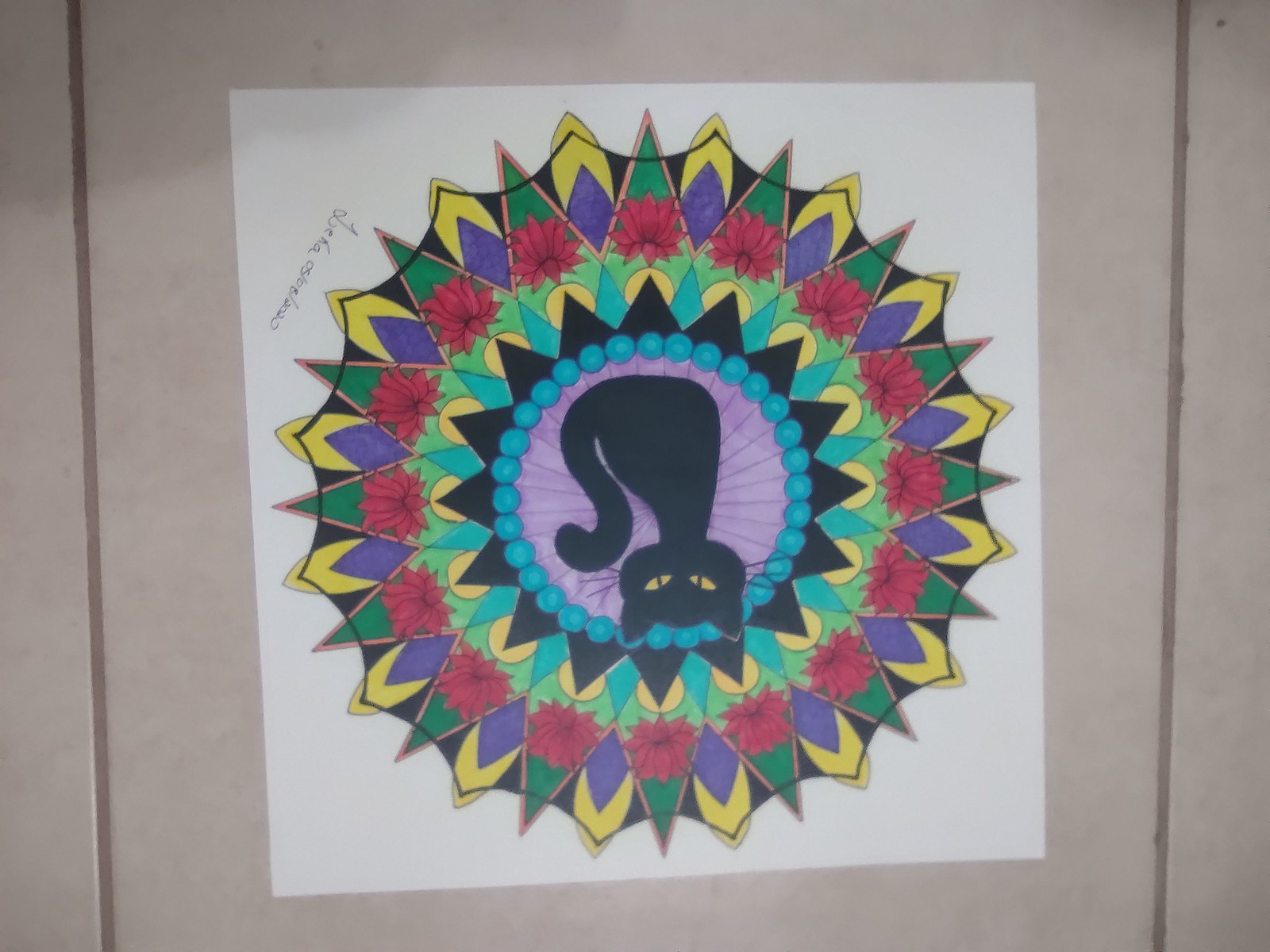This is an intricately detailed illustration on a white sheet of paper, positioned upside down against a grayish floor tile. At the center of the image is a black cat with vivid yellow eyes and black whiskers. The cat is encircled by a purple ring, which is adorned with a string of turquoise pearl-like beads. Surrounding this are black sun-ray-like triangles, which are intersected by a combination of triangles and circles, reminiscent of Pac-Man. This entire ensemble is engulfed in a kaleidoscopic pattern, featuring a starburst shape with intricate geometric shapes including blue triangles, yellow circles, and purple regions adorned with turquoise beads. The background features vivid red flowers with orange borders nestled within green triangles, all set against a patterned field of purple, yellow, green, and black. In the corners of each green triangle, yellow sunflower petals with blue diamond centers are interconnected by a black curve. The image also includes a signature, "Zika Ost Lobo 2020," positioned in what appears to be the upper left corner due to the upside-down orientation of the artwork. All of this is depicted against an off-white wall in the photograph.